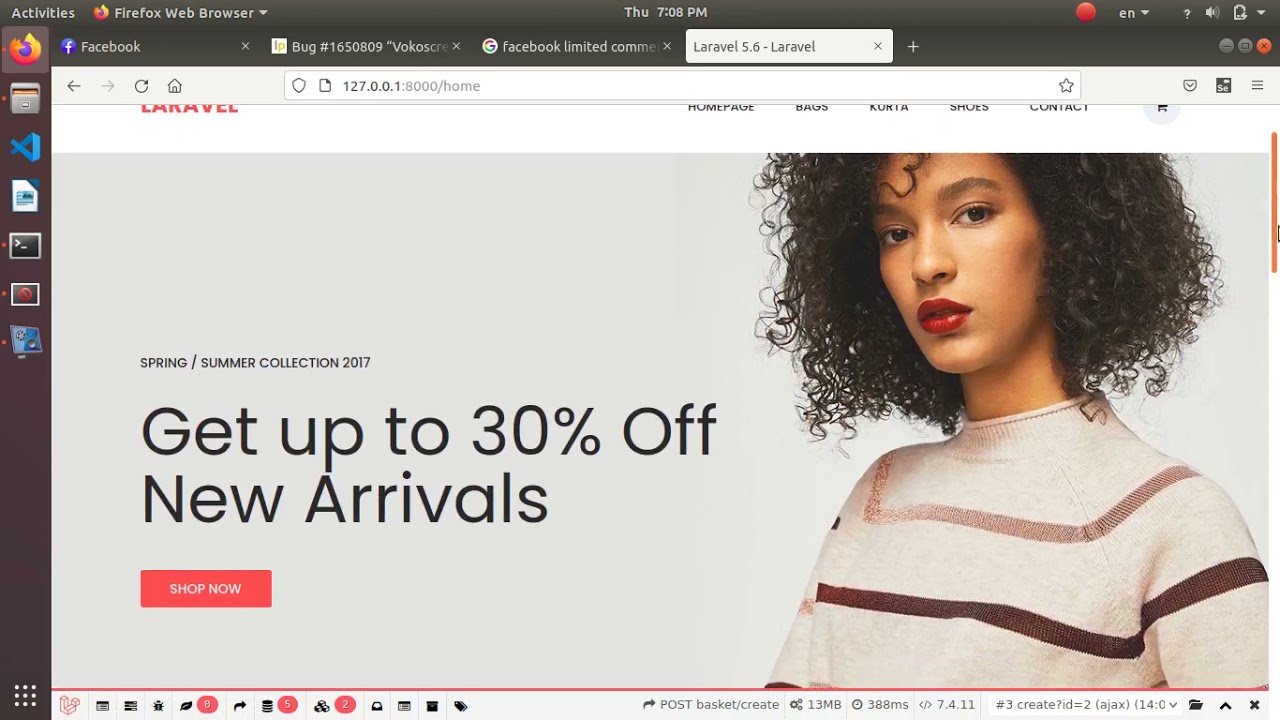The image appears to be a screenshot taken from a company's webpage, likely promoting a seasonal fashion collection. Dominating the center of the webpage is a high-quality photograph of an African-American woman, who is gazing stoically at the camera. She is adorned in a stylish sweater with tan, brown, and darker brown beige stripes. Her appearance is accentuated by her curly, brownish-black hair and vibrant red lipstick.

Overlaying the image, bold text reads "Get up to 30% off new arrivals," accompanied by a call-to-action button in a peachy-red color with white text that says "Shop Now." Above this, smaller text announces the "Spring/Summer Collection 2017." 

In one corner of the screenshot, you can observe that this is the fourth tab open in the browser. The other tabs include a Facebook page, a bug-related page, another Facebook page with limited comments, and possibly a Messenger tab. All these details highlight the promotional nature of the webpage currently being viewed.